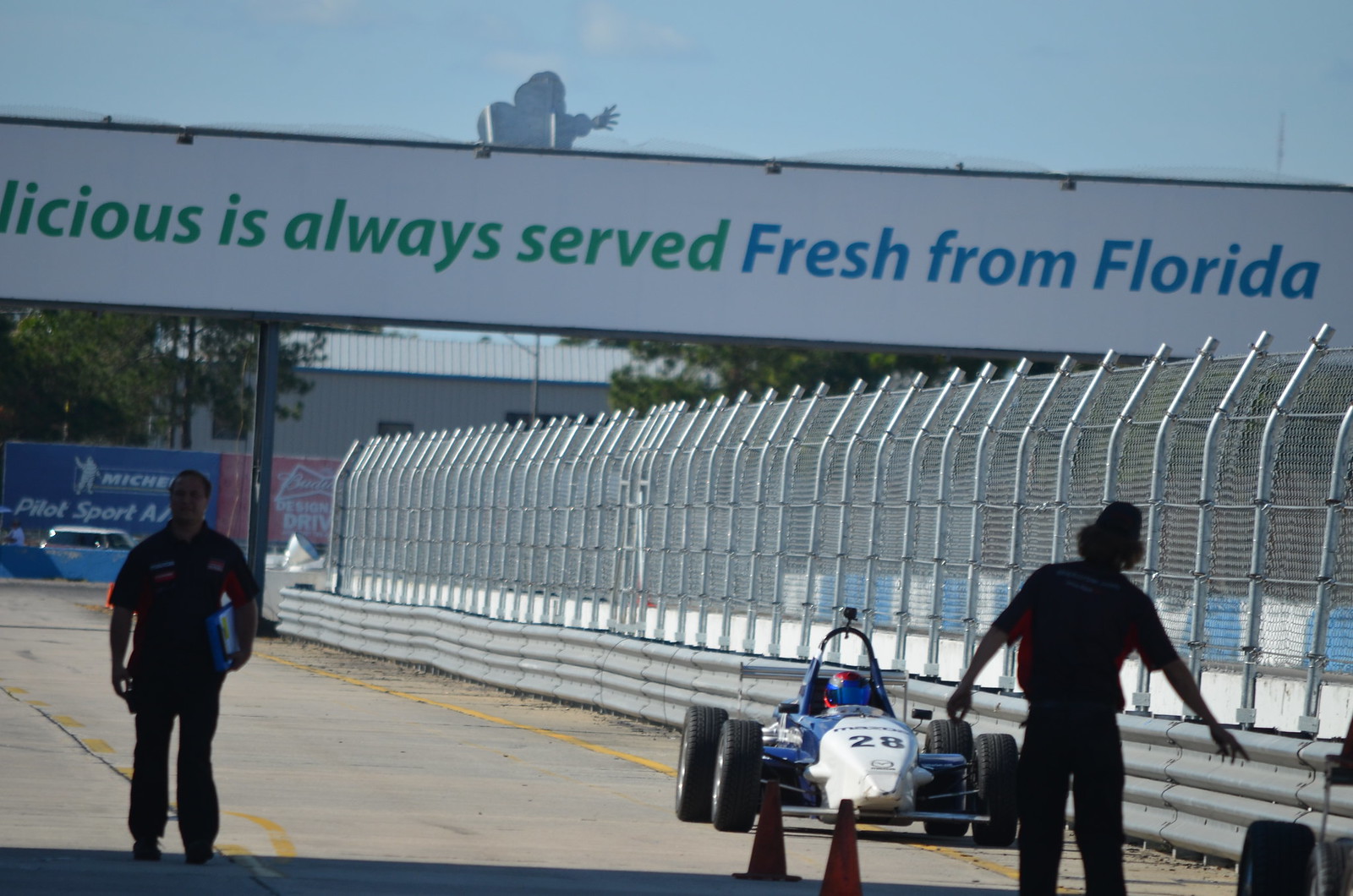The image captures a vibrant moment at a car racing event. Dominating the scene is a sleek blue and white race car numbered 28, driven by a helmeted driver, speeding towards a pit stop area marked by orange cones and yellow parking lines on gray pavement. Above the race track, a banner with green and blue text partially reads, "Licious is always served fresh from Florida," highlighted against a backdrop of clear blue skies and white clouds. In the foreground, two men are visible; one stands to the far left with long hair and his back to the camera, while another man in a uniform holds papers on the right side. Both appear to be part of the pit crew, ready for the incoming car. The scene is fenced off with a metal barrier, and various sponsor signs, including a blue one for Michelin Pilot Sport and a red one partially reading "drive," accentuate the event's atmosphere. In the deeper background, a float depicting a man, trees, and additional buildings add layers of depth to the bustling raceway environment.